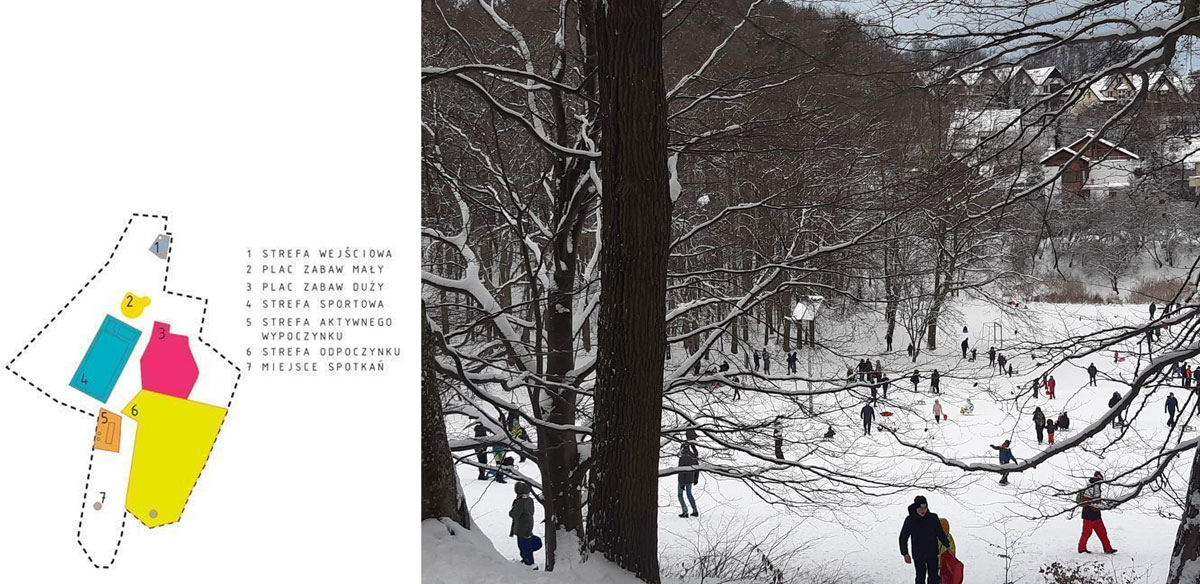The image captures a bustling winter scene at a ski resort. On the left side, there is a detailed map of the resort, adorned with various color-coded sections labeled in what appears to be Polish or another Eastern European language, detailing different areas numbered one through seven. Although the language is unfamiliar to observers, these sections include spots called "Strefa Wejściowa," "Plac Zabaw Mały," "Plac Zabaw Duży," "Strefa Sportowa," "Strefa Aktywnego Wypoczynku," "Strefa Odpoczynku," and "Miejsce Spotkań."

In the foreground, numerous people, bundled up in winter gear complete with coats, hats, and snow boots, are seen walking around, some carrying sleds. Notably, a man in a sled holds the hand of a child dressed in a yellow jacket and orange hat, and several individuals can be seen ascending towards the area on the right side of the image, suggesting the presence of a sledding hill.

The right side of the image showcases people actively moving about against a backdrop of what appears to be tightly-clustered houses, dusted with snow, and a snowy expanse extending further back, perhaps bordered by more trees or a mountain. The foreground is populated with snow-covered, leafless trees, adding a distinctively wintry ambiance to the scene. People appear to be enjoying various outdoor activities, contributing to the lively atmosphere of the ski resort.